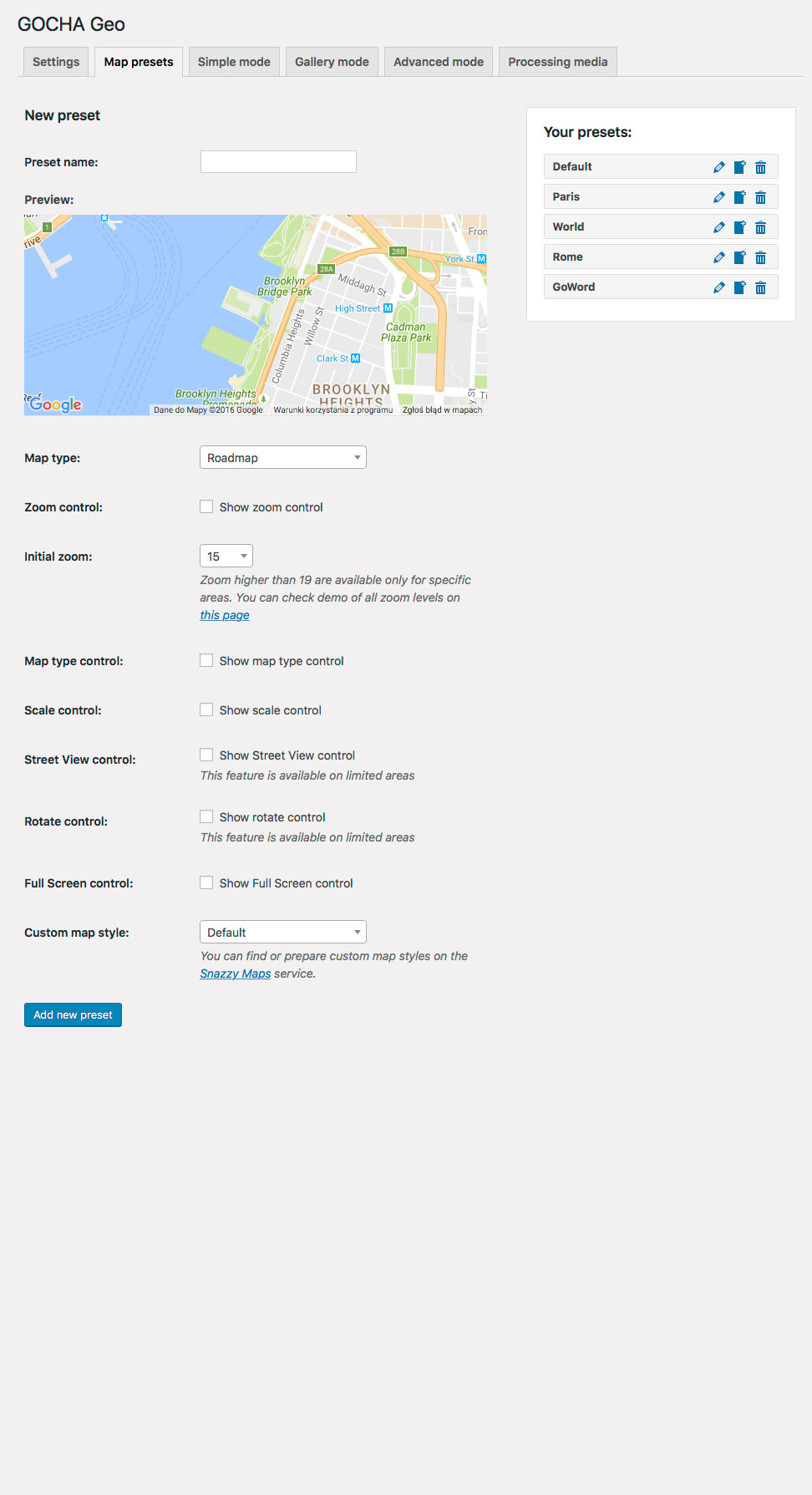This screenshot depicts a user interface with a predominantly white or gray background. At the top of the interface, there is a heading in all capital letters reading "GOCHA" (G-O-C-H-A). Below this heading, another label reads "GEL" (G-E-L), though the text is notably tiny, making it somewhat difficult to discern clearly.

The interface includes a selection of six tabs arranged horizontally. Among these tabs, two are specifically identifiable: one labeled "Settings" and another labeled "More places." The "Settings" tab is distinctly highlighted in black, while the remaining tabs feature gray text, blending subtly with the background. Additional tabs are labeled "New," "Preset," "Print," and "Name."

Below the tab navigation, the interface hosts a map centered on Brooklyn. Adjacent to the map, there are options to adjust map settings with labels that include "Map Type," "Zoom In," and other textual indicators that remain partially indistinct. Alongside, there is a list comprising four more items, enhancing the functionality and interactivity of the map. The specific details and inscriptions of these four items are currently unclear. 

Overall, this interface provides robust map-related functionalities with easy access to settings and navigation adjustments, all meticulously arranged for a user-centered experience.